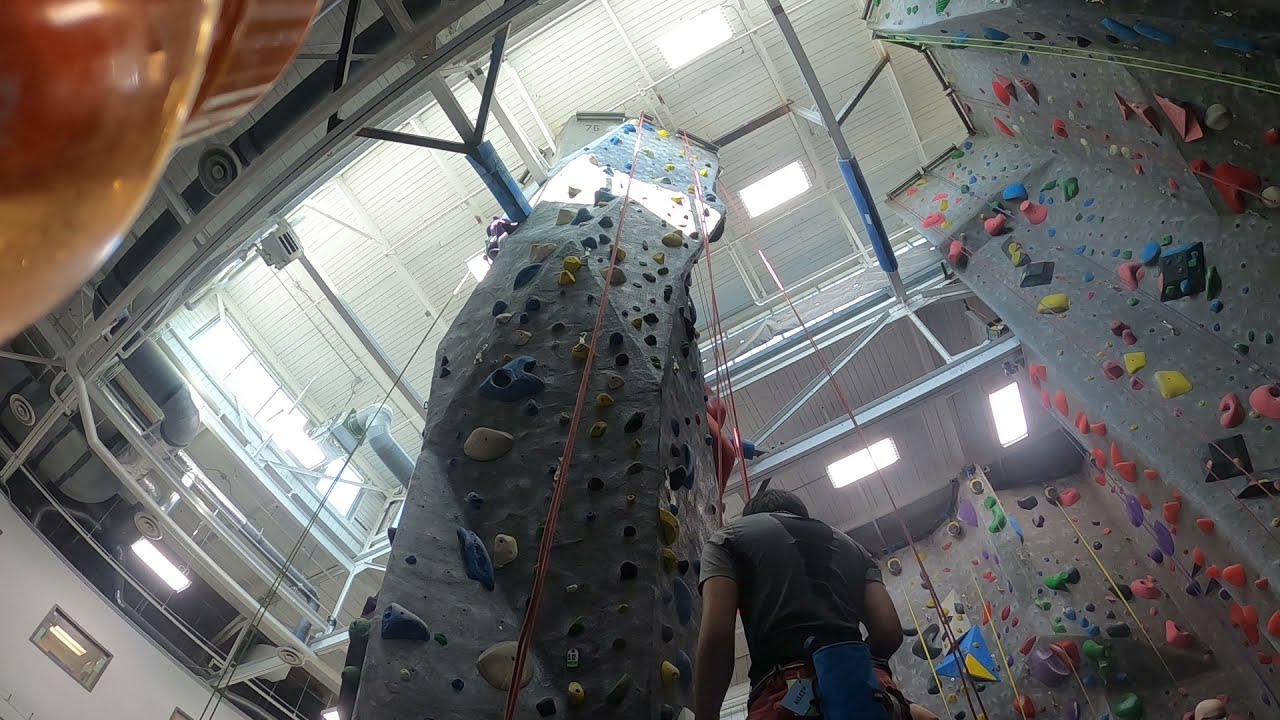This image captures an indoor rock climbing gym, featuring towering artificial climbing walls adorned with colorful handholds and footholds. The perspective is from the ground looking up, highlighting the height of the walls and the exposed rafters and corrugated ceiling above with lighting structures. A climber stands at the bottom center of the image, identifiable by his dark skin, reddish t-shirt, and climbing gear around his waist. He appears to be preparing for his ascent. Bright lighting, supplemented by natural light through a window on the left, illuminates the venue. Numerous ropes are in place from the top of these structures for safety, creating a secure environment for climbers to practice.